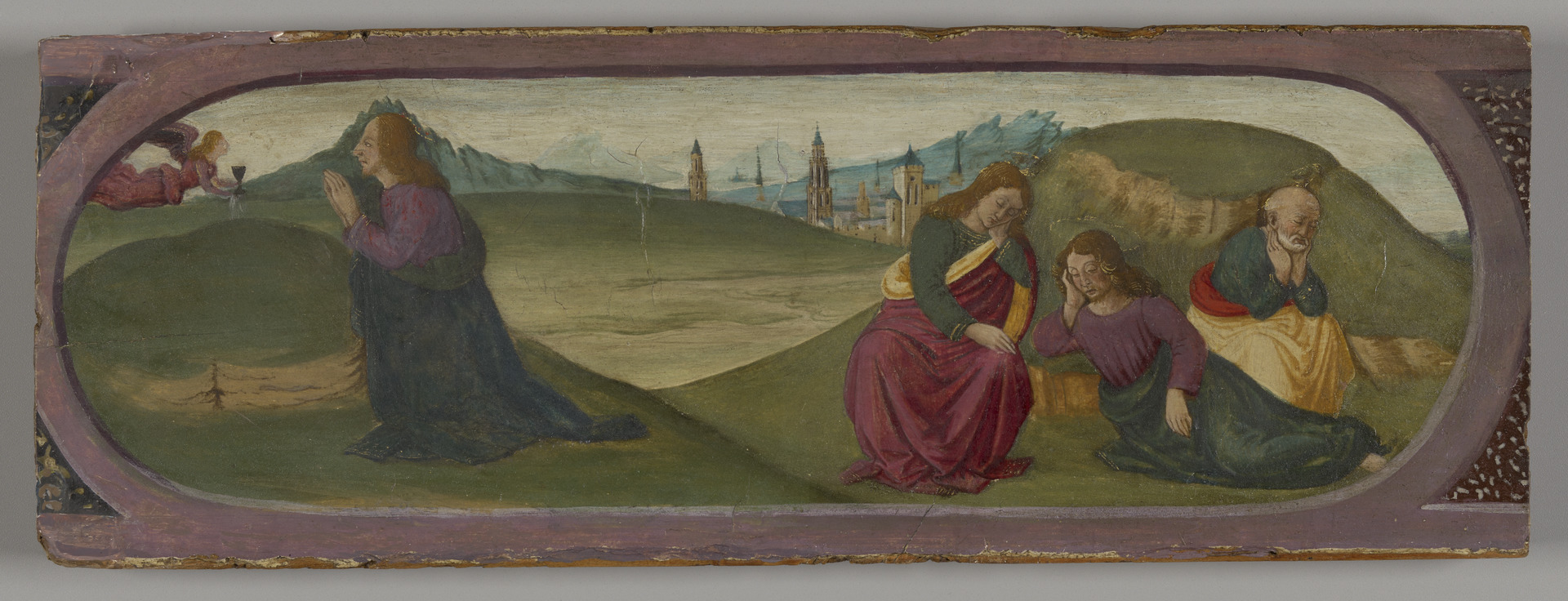This image appears to be a Renaissance-style painting on a rectangular wooden panel. The artwork, framed within an oval shape tinged with pink and purple hues, depicts a serene yet poignant scene. On the left, a woman in a posture of prayer is receiving a dark-colored glass, possibly containing wine, from an angelic figure. To the right, a small group comprising two young women in conversation and a solemn-looking man gazing down at the ground are gathered close together. They are adorned in bright, varied colors such as pink, green, red, purple, white, and yellow, suggesting their elevated status. Behind them, one can observe rolling hills and a distant cityscape featuring small towers and mountains, adding depth to the composition and evocative of an idyllic yet melancholic hillside setting. The absence of any text on the painting enhances its visual narrative.